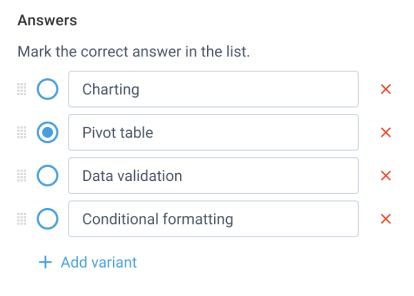The image appears to be a screenshot of a section of a website or an application interface. In the top left corner, the word "answers" is prominently displayed in bold, black text. Beneath it, in regular black text, is the instruction to "mark the correct answer in the list."

There are four selection options presented, each with a corresponding blue circle. The second option down has a blue dot in its center, indicating it has been chosen. Here are the four options listed in horizontal rectangles from top to bottom:

1. "Charting"
2. "Pivot Table" (selected)
3. "Data Validation"
4. "Conditional Formatting"

Each selection option also features a red "X" to its right. Towards the bottom of the image, there is a small blue plus sign followed by the words "add variant." Additionally, next to each blue circle on the left side of the options, there is a small grid of dots, four in total, representing draggable or interactive elements.

In summary, this interface allows users to select from a list of four options, with "Pivot Table" currently selected, as indicated by the blue dot within the corresponding blue circle.